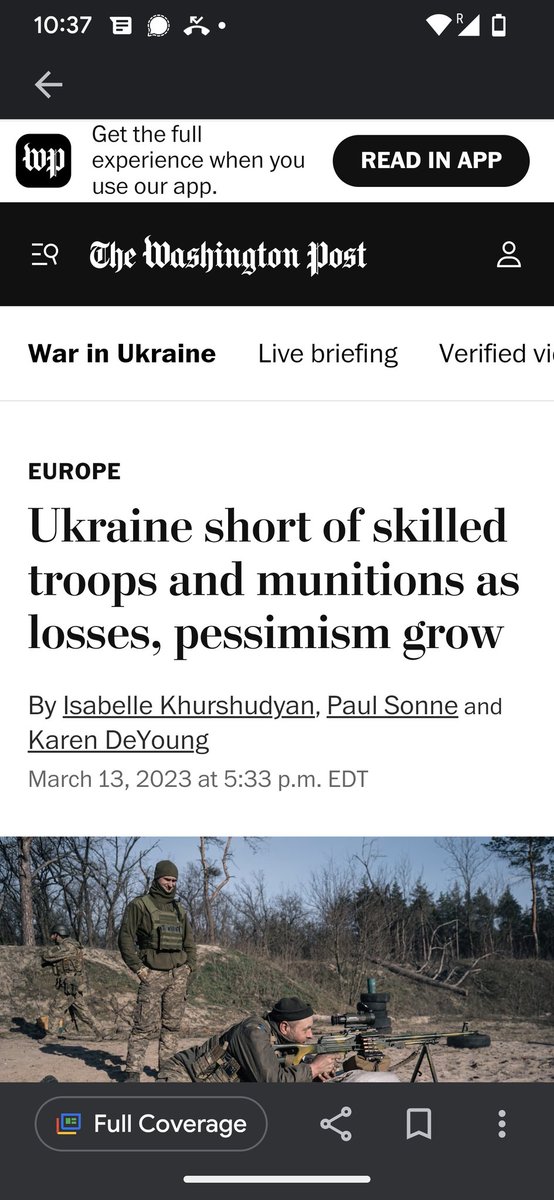Screenshot of a Washington Post news article taken on a smartphone. The time displayed at the top left corner is 10:37, and the battery level at the top right is less than one-fourth full. At the very top of the page, above the Washington Post logo, there is an advertisement for the Washington Post app, which reads, "Get the full experience when you use our app." To the right of this statement, there is a link labeled "Read in app," and on the left side, the app's logo is shown, simply marked as "WP."

The Washington Post banner is black with the publication's name in white text. Directly below the banner are navigational tabs. The visible tabs from left to right are "War in Ukraine," "Live Briefing," and partially obscured tabs. The "War in Ukraine" tab is highlighted in dark black text, indicating the current section being viewed.

Beneath these tabs is a section labeled "Europe," followed by the headline of the featured article: "Ukraine short of skilled troops and ammunitions as losses, pessimism grows." The byline lists the authors of the article: Isabel Khurshudyan, Paul Sonne, and Karen DeYoung.